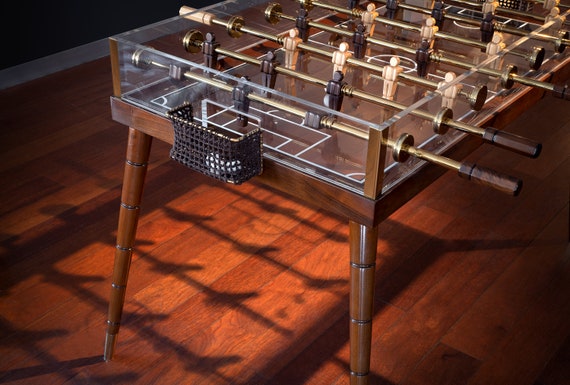This close-up image showcases an elaborate and elegant foosball table situated on warm, dark red hardwood floors. The table features unique long, dark brown wooden legs with cylindrical silver accents at the bottom. The table's sides are constructed from thick, clear acrylic, giving it a sleek and modern look. The playing field of the foosball table is also made of clear acrylic. The handles, wrapped in dark brown leather, add a sophisticated touch while the small foosball players are colored in black, white, and shades of brown and tan. Each end of the table features a rectangular metal goal net with a black mesh. The ambient lighting creates a shadow beneath the table, adding depth to the image, and part of a wall can be seen in the top left-hand corner, contributing to the room's cozy setting. The foosball table is clearly the central focus, emphasized by the detailed craftsmanship and materials used in its design.